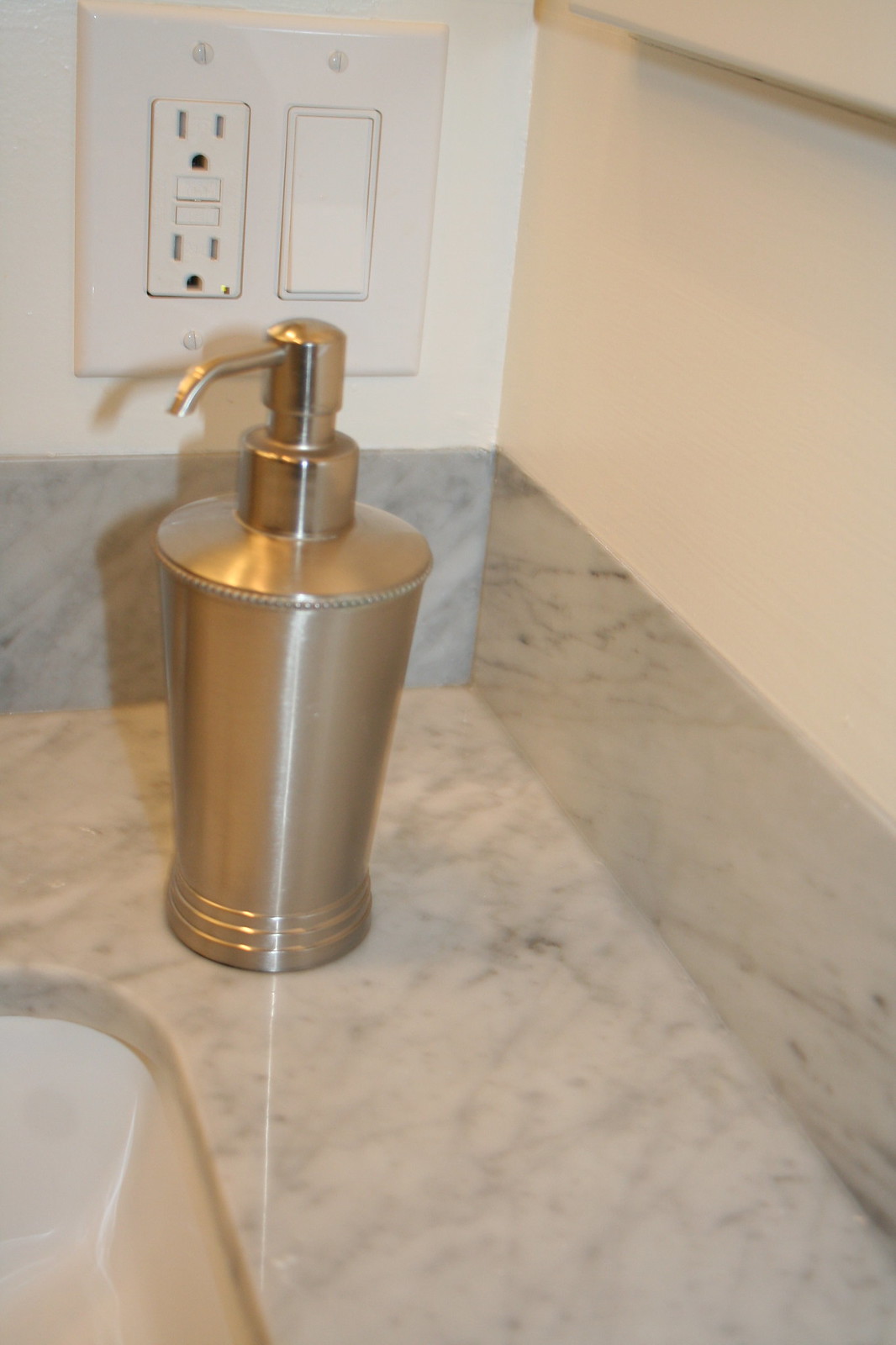The image captures a detailed close-up corner of a sink embedded in a marbled countertop. The countertop is light gray with subtle black veining, lending it a sophisticated yet understated appearance. The sink is positioned adjacent to a white-painted wall, which features a pair of electrical outlets and a light switch situated just above the sleek golden metal container meant for holding liquid soap. The vibrant sheen of the gold container juxtaposes the cool tones of the marble and the wall, drawing the eye. In the upper right corner, part of a frame is visible, suggesting the presence of a towel rack nearby. The overall arrangement and choice of materials evoke a modern, elegantly functional design aesthetic.